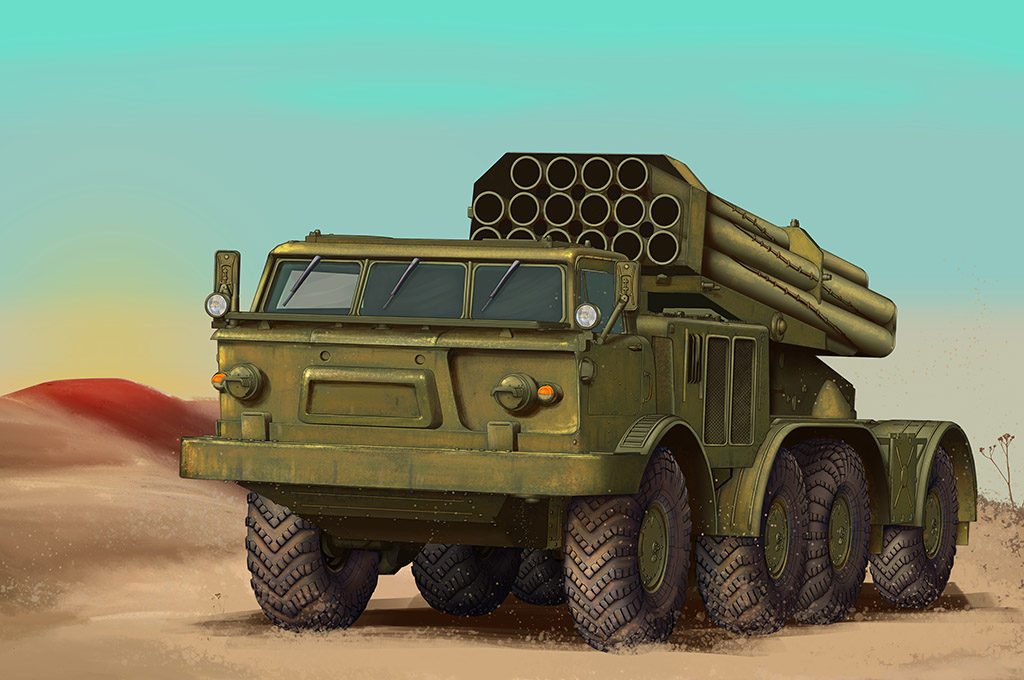This digital artwork, framed in a horizontally oriented rectangle, depicts a military scene set in a vast, flat desert environment under a blue sky. The sky, painted in turquoise hues with subtle purplish-gray clouds and a hint of a yellowish sun peeking through on the left, stretches above a sandy, tan ground with sparse, scrubby vegetation visible in the background to the right. Dominating the scene is a large, olive green military vehicle, identifiable as a tank or truck, equipped with eight sizable wheels, four on each side. The vehicle's broad windshield is divided into three segments, each fitted with a windshield wiper. Mounted on the back of the vehicle is an imposing multi-missile launcher system with space for sixteen rockets, arranged in two lower rows of six tubes each, topped by a single row of four tubes. Subtle red accents, possibly control knobs, are visible near the front of the vehicle, contrasting against its overall army green color.